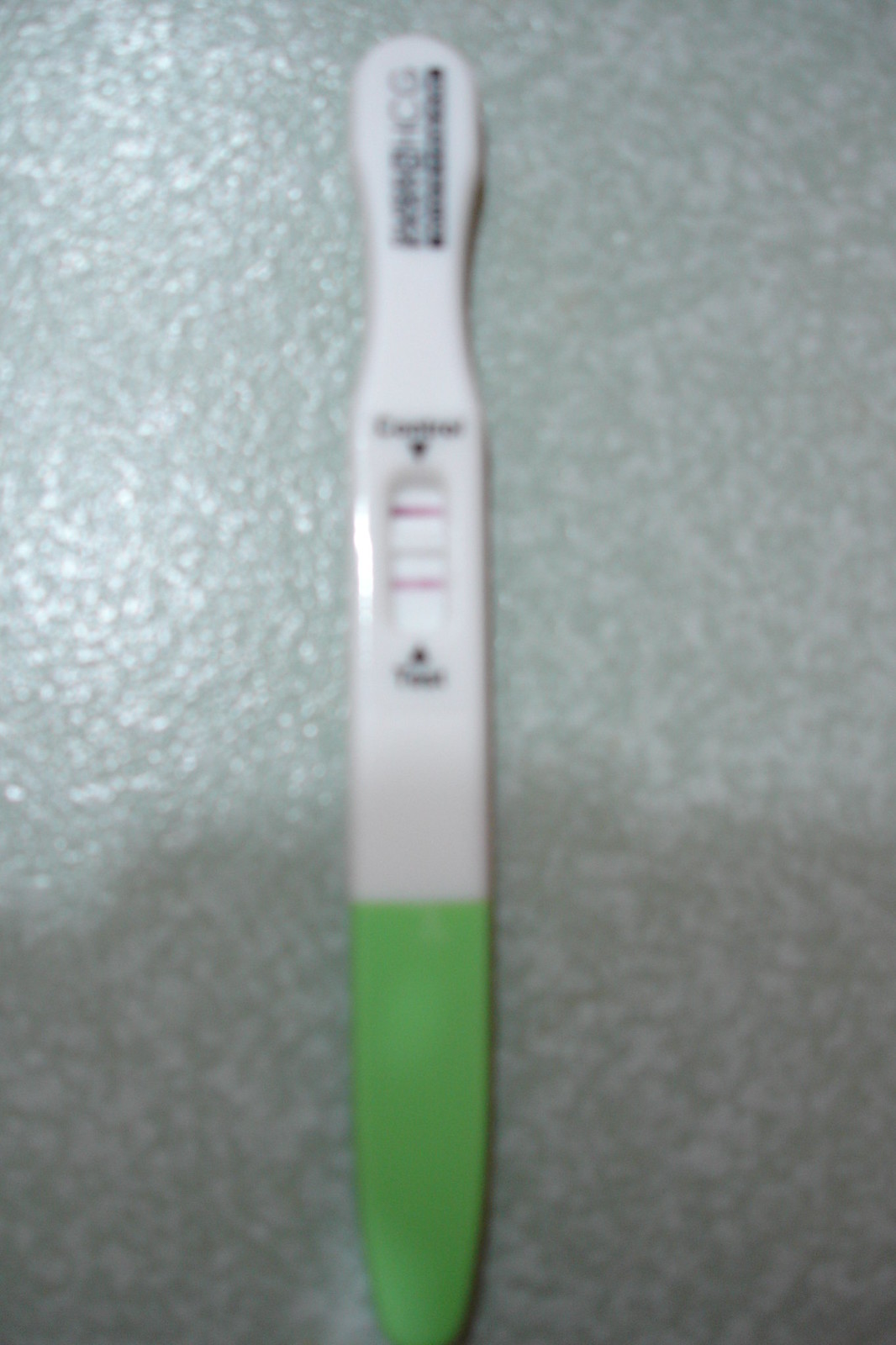The blurry image showcases a dipstick test strip encased in a holder, set against a modeled pale gray and medium gray background. The holder bears a resemblance to a stretched-out hourglass or the shape of a toothbrush, particularly in the section above the test strips where it curves inward and then flares out slightly. The bottom portion of the dipstick holder is lime green, transitioning into a white center section that houses detection strips visible through a small window. The two horizontally-aligned red lines on the white strips are separated by a space, suggesting the presence of two distinct test areas. This white section also features black writing above and below the test strip window, with the upper text accompanied by a downward-pointing arrow and the lower text by an upward-pointing arrow. At the top of the holder, where the white section is cut off in the image, vertical black text is visible but not legible. The lighting in the image casts a shadow along its bottom third, while a reflection is noticeable on the upper left side, giving the impression that the light source is stronger in this area. The white portion of the holder extends slightly outside the frame, suggesting a rounded end.